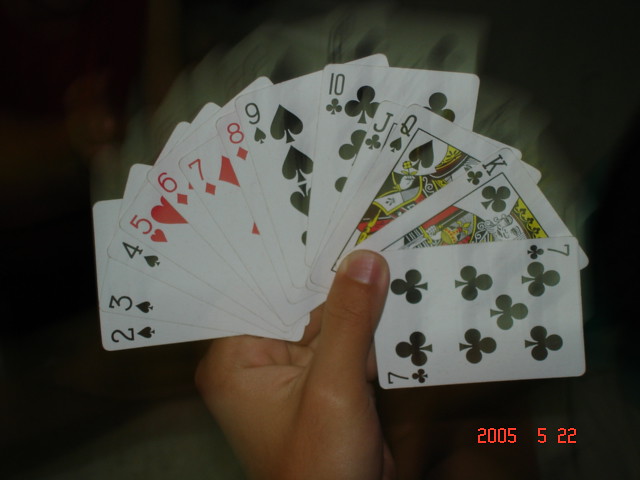A person is holding a fan of playing cards, seemingly poised to play a card game. The image was captured with a regular camera, and in the bottom right corner, a digital timestamp in red reads "2005 5 22." The cards in the person's hand are slightly blurred, as if motion was captured, creating a ghostly, translucent effect of an additional row of cards above the primary set. The visible cards, from left to right, are a 2 of Spades, 3 of Spades, 4 of Spades, 5 of Hearts, 6 of Diamonds, 7 of Diamonds, 8 of Diamonds, 9 of Spades, 10 of Clubs, Jack of Clubs, Queen of Spades, King of Clubs, and a 7 of Clubs. The background is a deep and uninterrupted black, offering stark contrast to the vibrant and dynamic arrangement of the cards.